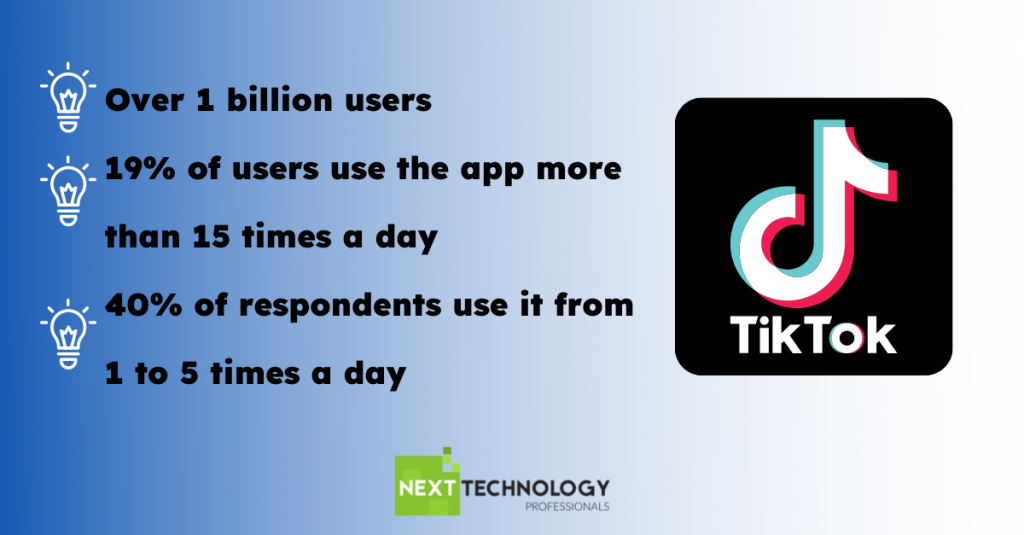The image features a horizontal, rectangular design with a blue gradient background. This gradient transitions from a solid medium blue on the left to a bright white on the right. Dominating the right side of the image is a large black box that houses the TikTok logo. The logo itself is white and is outlined with blue and pink accents, making it pop against the black backdrop.

Aligning the left edge of the black box is a set of three white lightbulb icons, each serving as a bullet point for the black text to their right. The text includes the following statistics: 
1. "Over 1 billion users."
2. "19% of users use the app more than 15 times a day."
3. "40% of respondents use it from 1 to 5 times a day."

At the very bottom center of the image is a green rectangle with the word "NEXT" written in white capital letters. Positioned just to the right of this green rectangle is the black text reading "Technology Professionals," which together forms the term "Next Technology Professionals".